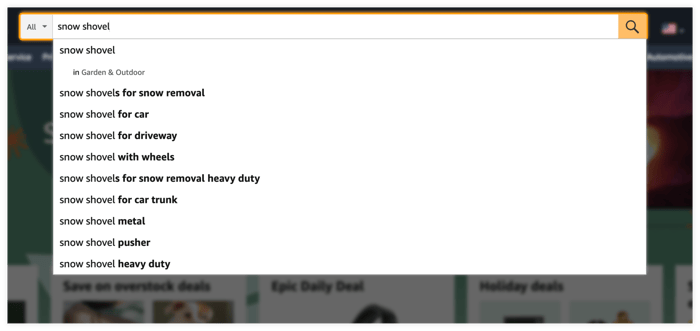The image is a screenshot of an Amazon search bar displaying the query "snow shovel." Below the search bar, a list of auto-complete suggestions related to the search term is visible. The first suggested search is simply "snow shovel," categorized under "Garden and Outdoor." The subsequent suggestions include "snow shovels for snow removal," "snow shovel for car," "snow shovel for driveway," "snow shovel with wheels," "snow shovels for snow removal, heavy duty," "snow shovel for car trunk," "snow shovel metal," "snow shovel pusher," and "snow shovel heavy duty." The background of the image is slightly blurred, featuring additional recommended items typically seen on Amazon's interface.